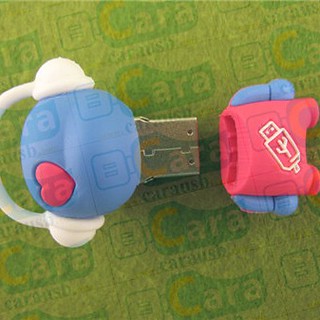This image depicts a whimsical USB flash drive designed to resemble a small toy figurine, set against a vibrant lime green background adorned with the word "Kara" in a bubbly font. The left side of the USB drive forms the head of the character, which is a rounded blue shape adorned with a pink heart where the left eye might be. The head is topped with white earmuffs, adding to its playful design. On the lower part of the head, a metallic USB connector protrudes, clearly indicating its function as a flash drive. 

The body of the character, which serves as the cap for the USB drive, is a pink and purple section that fits over the USB connector. This section comprises the figurine's torso and arms. Notable details include the white emblem on the character's chest, resembling a small USB drive illustration, and the intricate design components such as the overall color contrast and thematic elements that blend the appearance of a toy with practical tech functionality. The visual harmony of the USB device with its colorful and imaginative design makes it an eye-catching and unique gadget.